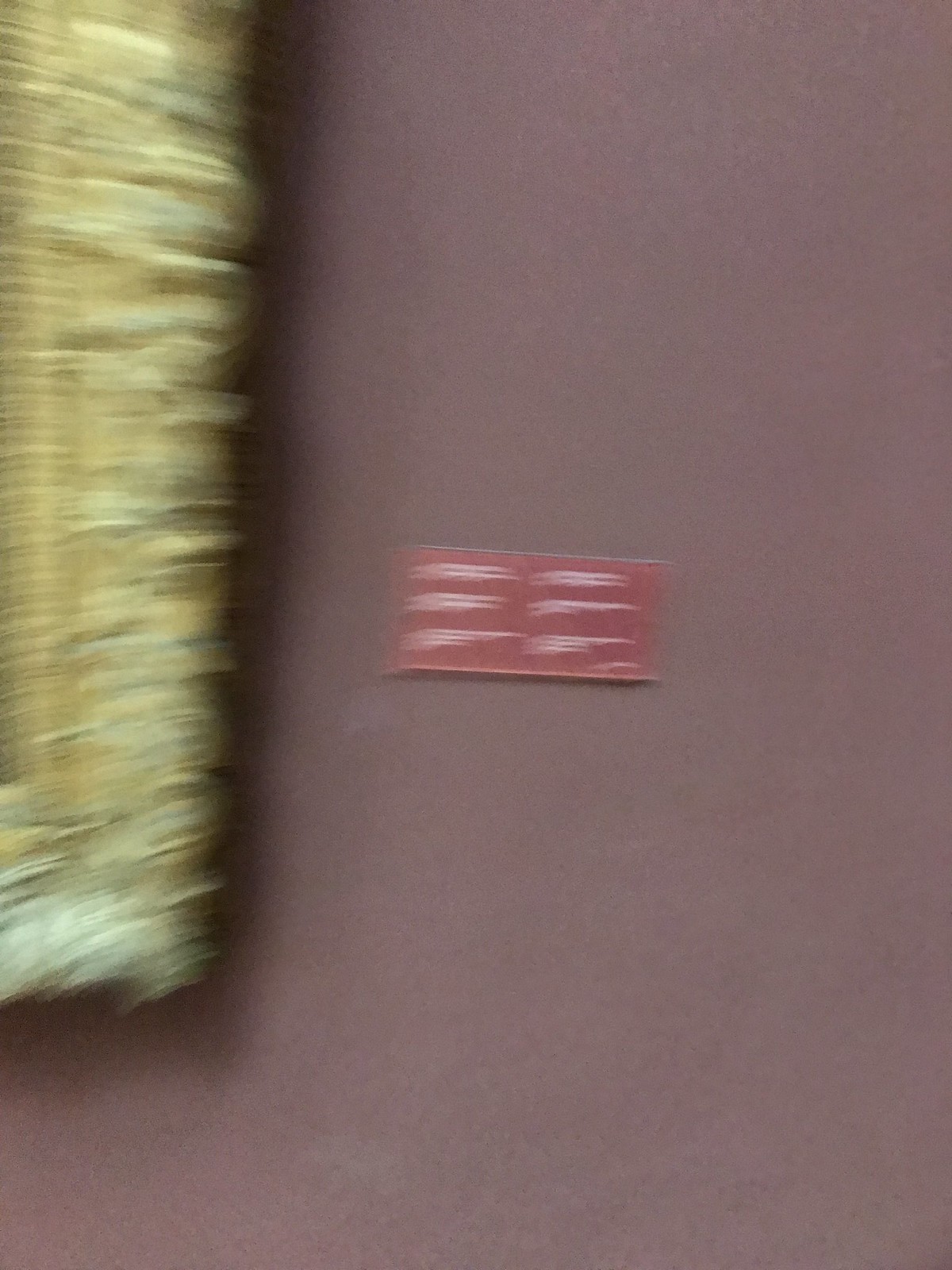In this image, a portion of a wall can be seen, adorned with a meticulously constructed golden frame. The craftsmanship of the frame is evident despite the slight blurriness and shakiness of the picture. The golden frame features intricate details that suggest a high level of artistry; however, it's unclear whether the frame is genuinely made of gold or simply painted to achieve that effect. Only the right side of the frame is visible, and its full length is not captured within the shot. Adjacent to the frame, there is a red plaque that provides detailed information about the artwork, including its history, the artist's identity, the creation process, and the inspiration behind it. Unfortunately, these specific details remain unreadable due to the distance and blurred quality of the image. The wall itself is colored in a dusty rose or brownish hue, providing a warm backdrop that complements the framed piece and the informational plaque.